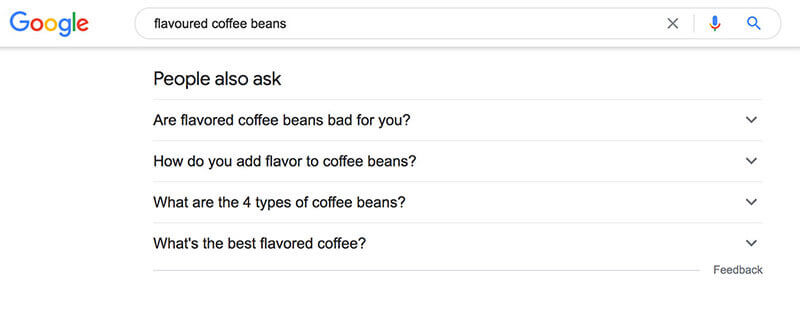Here is a detailed descriptive caption:

"The image is a screenshot of a Google search query page. At the top left, the iconic Google logo is prominently displayed, featuring its characteristic letters in blue, red, yellow, and green. Below the logo is a search bar, currently displaying the query 'flavored coffee beans,' followed by an 'X' icon to clear the text, a colorful microphone icon in blue, red, yellow, and green for voice search, and a blue search button icon. 

Underneath the search bar, in large black letters, the text 'People also ask' is shown, accompanied by four related questions: 

1. 'Are flavored coffee beans bad for you?'
2. 'How do you add flavor to coffee beans?'
3. 'What are the four types of coffee beans?'
4. 'What's the best flavored coffee?'

Each question is listed on a separate line and features a small downward-facing arrow on the right-hand side, indicating that additional information can be expanded for each query. The background of the entire page is a plain white, creating a clean and minimalistic look."